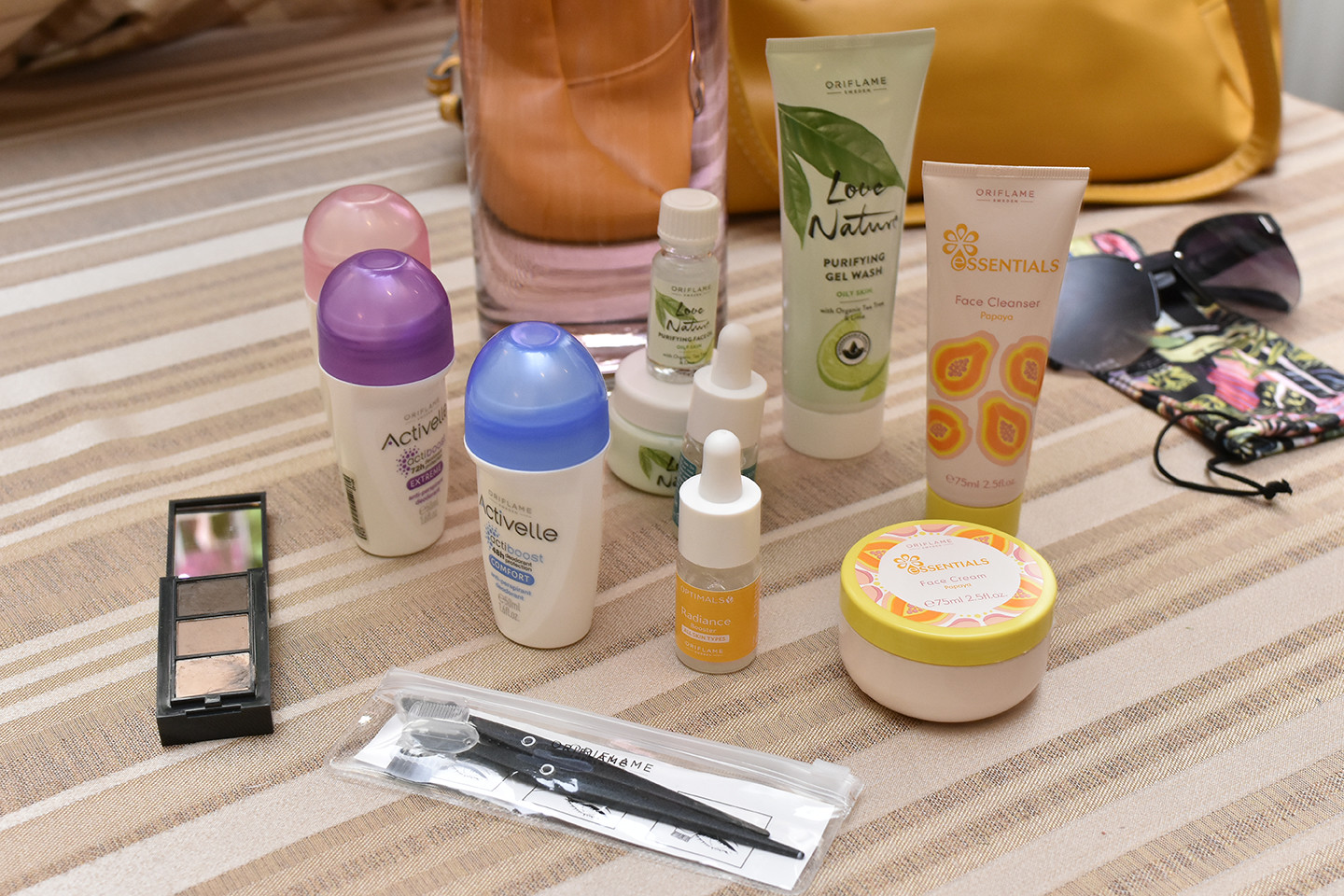The photograph showcases a variety of cosmetics arranged on a striped cloth, featuring tan, white, and a hint of brown. The background includes an orange pocketbook partially visible at the top, with the bottom half prominently displayed. Below and to the right of the pocketbook, a pair of sunglasses rests atop a floral-printed sunglass holder. To the left, several moisturizers are lined up, including a green tube and a white tube, accompanied by additional bottles with pink, purple, and blue caps. A couple of smaller, eyedrop-style containers are also present. On the far left, an eyeshadow palette with three different shades is visible, and in the bottom portion of the image, a set of brushes in a small case, likely for applying the eyeshadow, is displayed. Overall, the image portrays an assortment of moisturizers, lotions, and makeup products.